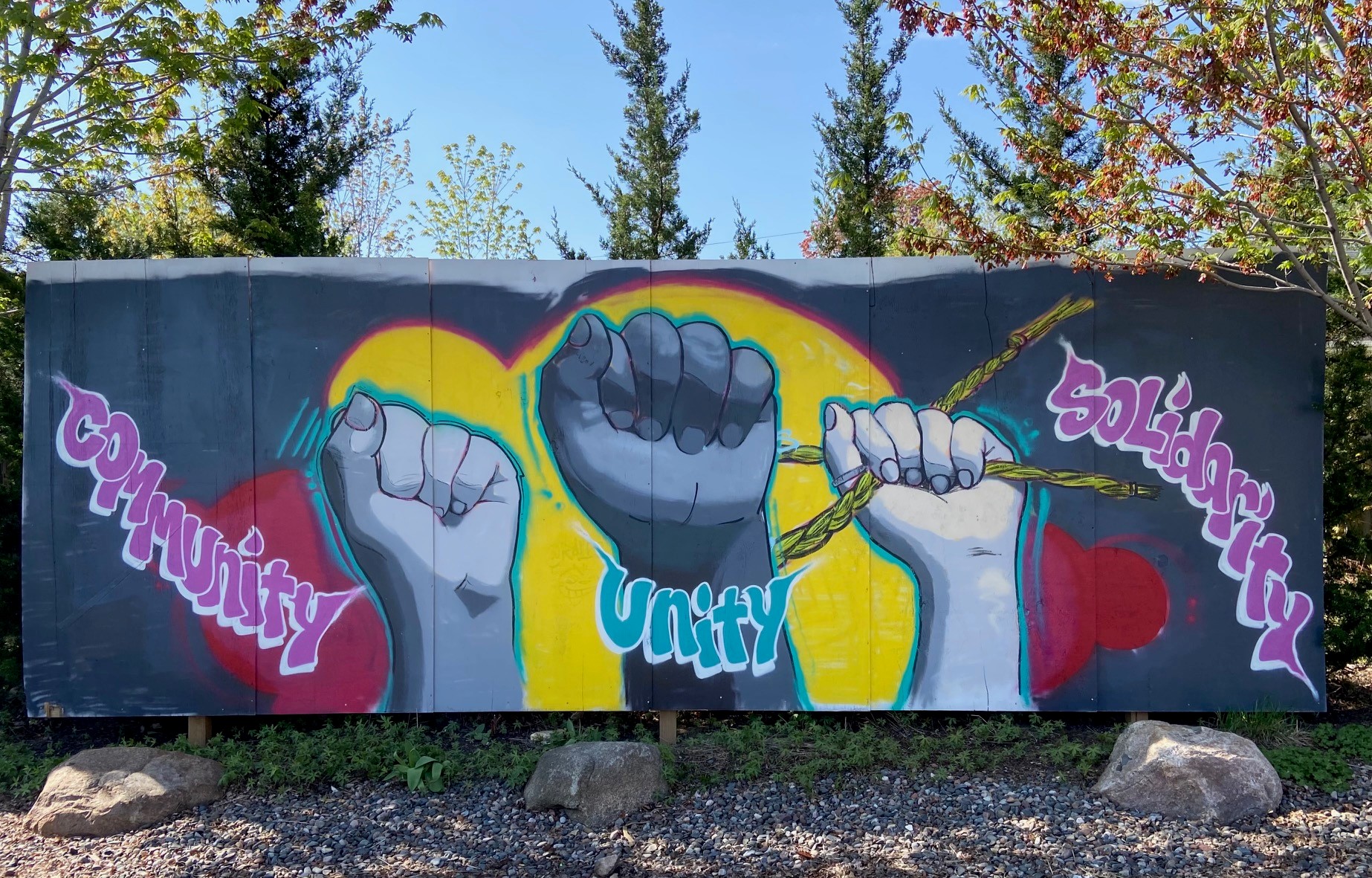In front of a lush, forested area with a mix of tall green pine trees and deciduous trees turning their fall colors, there stands a large, rectangular bulletin board, erected by three wooden posts. Beneath this board, positioned at even intervals, are three substantial gray boulders set on a light gravel road composed of gray and dark gray stones. The board itself is spray-painted gray and prominently features striking graffiti artwork. 

At the center of the board is a black or dark gray fist, surrounded by a vibrant yellow heart with red blobs on either side. On this central fist, the word "Unity" is written in an aqua blue color. Flanking this central image are two white or light gray fists. The left fist is paired with the word "Community" in purple text, while the right fist, which holds two peculiar ropes or strings, is accompanied by the word "Solidarity," also in purple text. This detailed and colorful mural encapsulates the themes of unity, community, and solidarity against a serene natural backdrop.